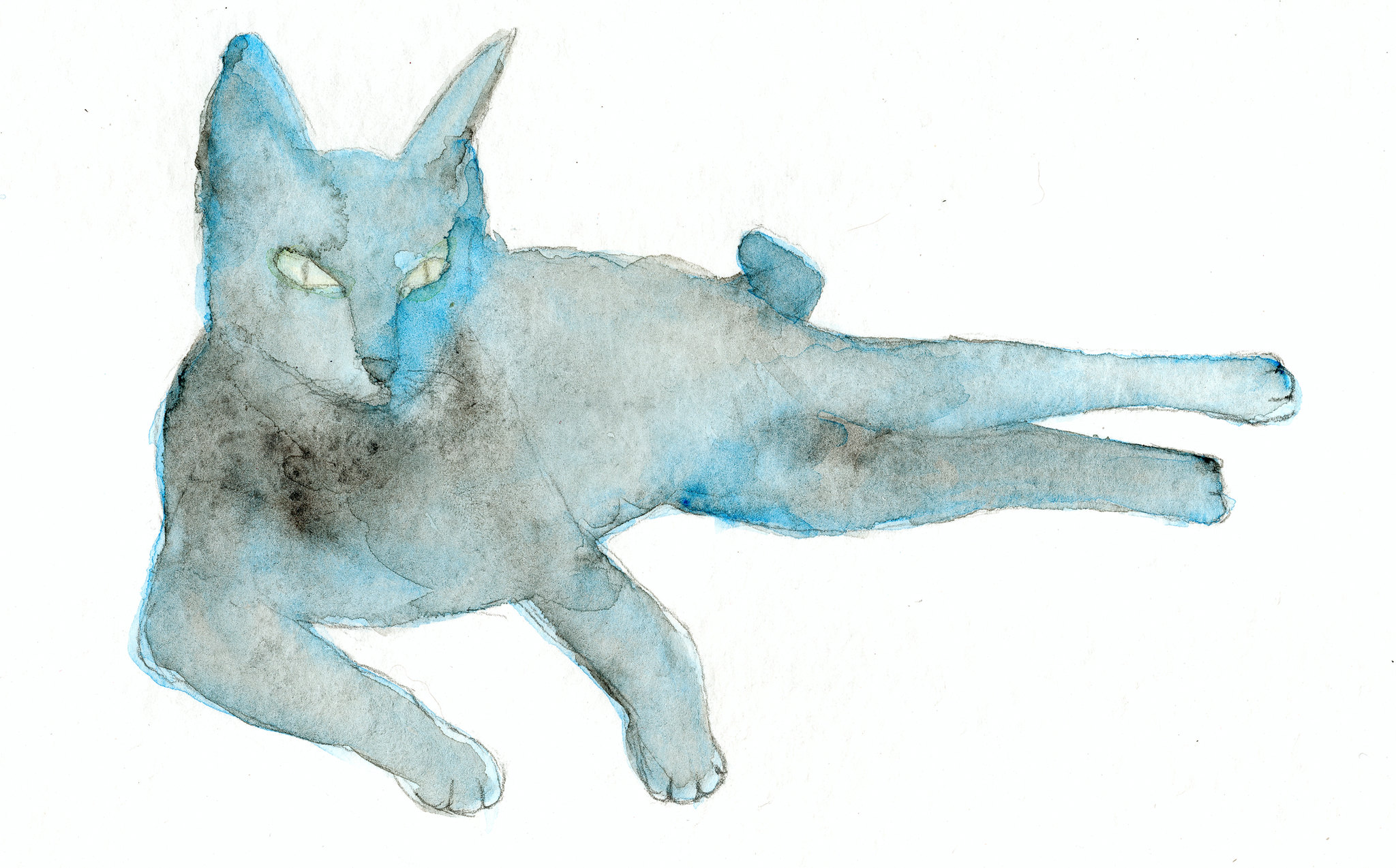This rectangular image, set against an all-white background, features a watercolor painting of a cat using primarily shades of blue, white, and touches of black. The cat, stretched out on its side with its head to the left and hind legs extended to the right, is depicted in a unique blend of light blue and white with hints of black, giving it an overall light gray tone. Various parts of the cat, such as its tail, legs, and face, have concentrated blue hues, creating a striking contrast. The cat's eyes are a very light color, almost white with a hint of yellow and detailed gray-blue irises with slit pupils. It has perky ears, a small black nose, and visible black whiskers. The chest area is shaded darker, achieved by layering brown tones to almost black. The forearms are stretched out, with the right one bent slightly. Look closely and you’ll notice the tail is nearly hidden, appearing as a small nub in the background.